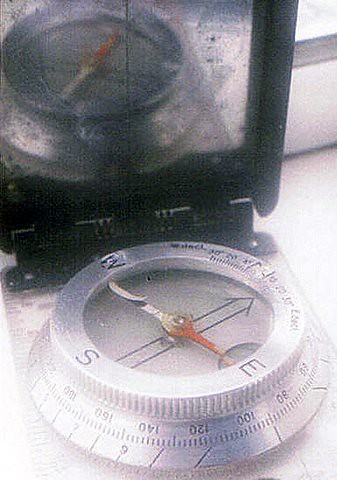This photograph, albeit of not very high resolution, captures a round metal compass in either a silver or gray hue. The compass dial is prominently marked with the letters "E," "S," and "W" among other indistinguishable letters. An orange and silver hand points within the compass, accompanied by a black outlined arrow on its face. Surrounding the rim of the compass are black letters, though their specific content remains unreadable.

The base of the compass is adorned with numbers including 100, 120, 140, 160, 180, and possibly 80, with small hash marks situated beneath these numbers. Additionally, diagonal lines and numerals "9" and "7" are present. The compass is placed upon a white base.

In the foreground, a computer monitor or display is visible. This monitor shows a blurred image of a similar-looking compass where the needle points elsewhere. This display is encased in a black frame.